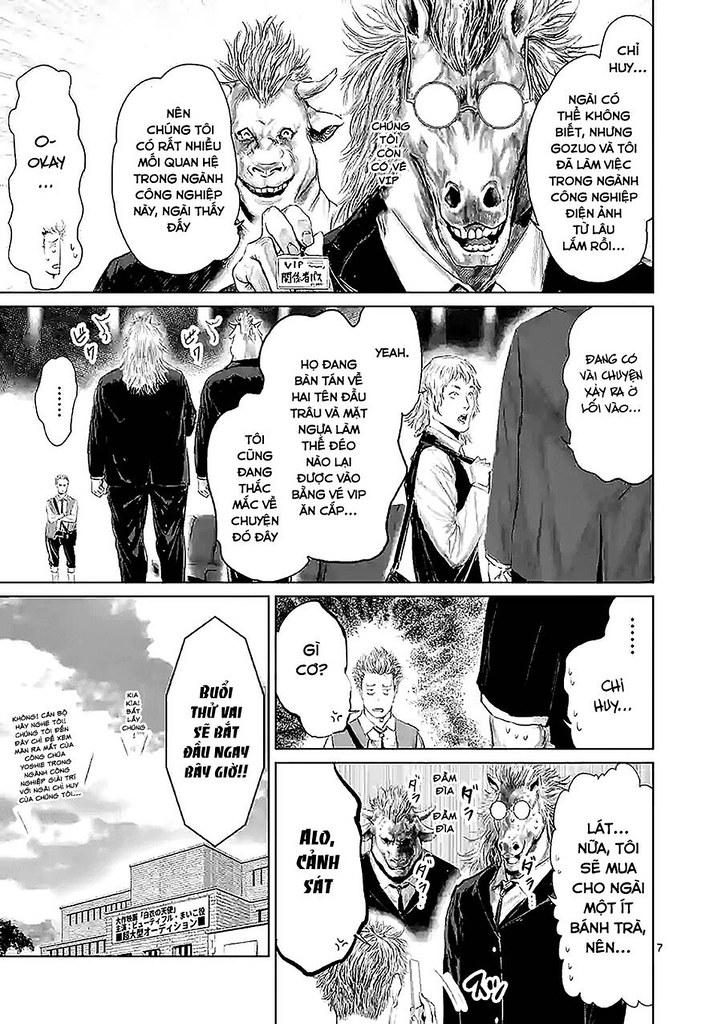The image is a black-and-white comic strip in the Eastern manga style, depicting a scene across five detailed panels. The top portion of the strip consists of two stacked panels, followed by three panels at the bottom—one on the left and two on the right. The comic features humanoid characters with animal heads, including a horse-headed individual with glasses and a VIP badge, dressed in a suit, and a pig-headed individual in similar attire. There is also a mention of a bull-headed character with spiked hair. 

In the first panel, the horse-headed and pig-headed characters are engaged in a conversation. The subsequent panels show the backs of these anthropomorphic figures interacting with other characters, some of whom appear to be ordinary humans. The dialogue is in a non-English language, possibly Vietnamese, and the scene suggests a confrontation is brewing but not fully realized within these panels. There is a brick building in the background of the bottom panel, adding to the detailed setting. The comic is noted for its intricate and well-drawn style, capturing various conversations through speech bubbles.